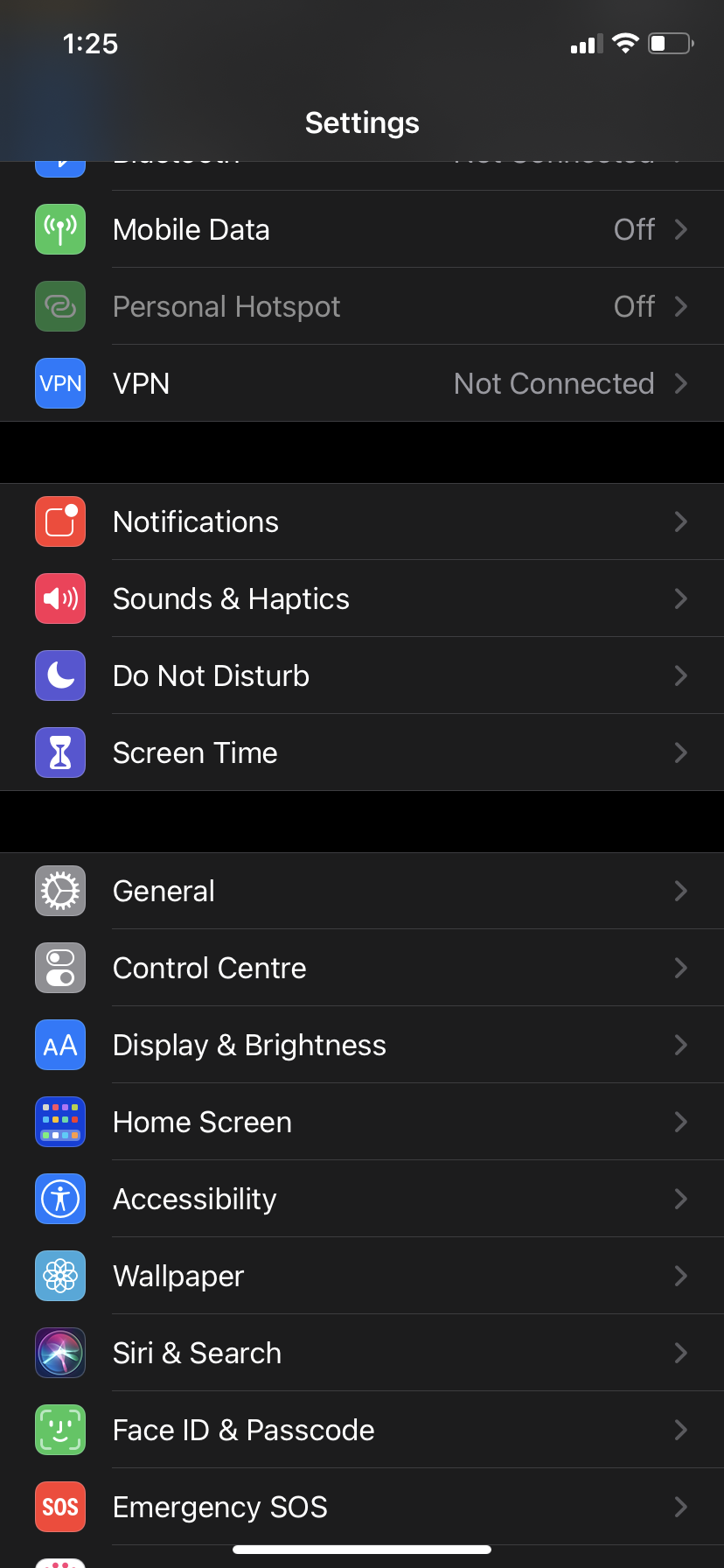The screenshot captures an iPhone's "Settings" menu, featuring a comprehensive list of various configuration options. At the top, "Mobile Data" is listed, followed by "Personal Hotspot," which allows users to share their cellular connection. "VPN not connected" indicates the device currently isn't using a Virtual Private Network. The "Notifications" section is visible for managing app alerts, along with "Sound & Haptics" to adjust audio and vibration settings.

"Do Not Disturb" can be seen for silencing notifications, and "Screen Time" helps monitor and manage device usage. "General" includes broader settings, while "Control Center" offers quick access to essential functions. "Display & Brightness" allows adjusting screen preferences, and "Home Screen" customizes app arrangement and appearance.

"Accessibility" appears prominent for users needing special accommodations, and "Wallpaper" provides options for background customization. "Siri & Search" configures the virtual assistant's behavior. Finally, "Face ID & Passcode" enhance device security, and "Emergency SOS" settings are available for urgent situations.